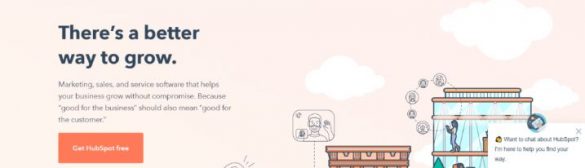The header of the website for a marketing service company features a serene background comprising a pink sky with scattered clouds on the right side. On the left side, in bold black lettering, the tagline reads, "There's a better way to grow." Below this, a subheading elaborates, "Marketing, sales, and service software that helps your business grow without compromise," followed by the quote, “Good for the business should mean good for the customer.”

Underneath this text, a red rectangular button with white lettering offers a call to action: "Get HubSpot Free," serving as a link. 

On the right side of the header, the visual elements include illustrations of two buildings. In the upper section of the rightmost building, a woman appears to be engaged on her phone, with a circle emanating from her, displaying various contact images. Near the other building, an illustration of a person smiling and with their arm raised, as if video chatting, can be seen. 

In the bottom right corner, a link reads, "Want to chat about HubSpot? I'm here to help you find your way," inviting users to initiate a chat with a bot on the website.